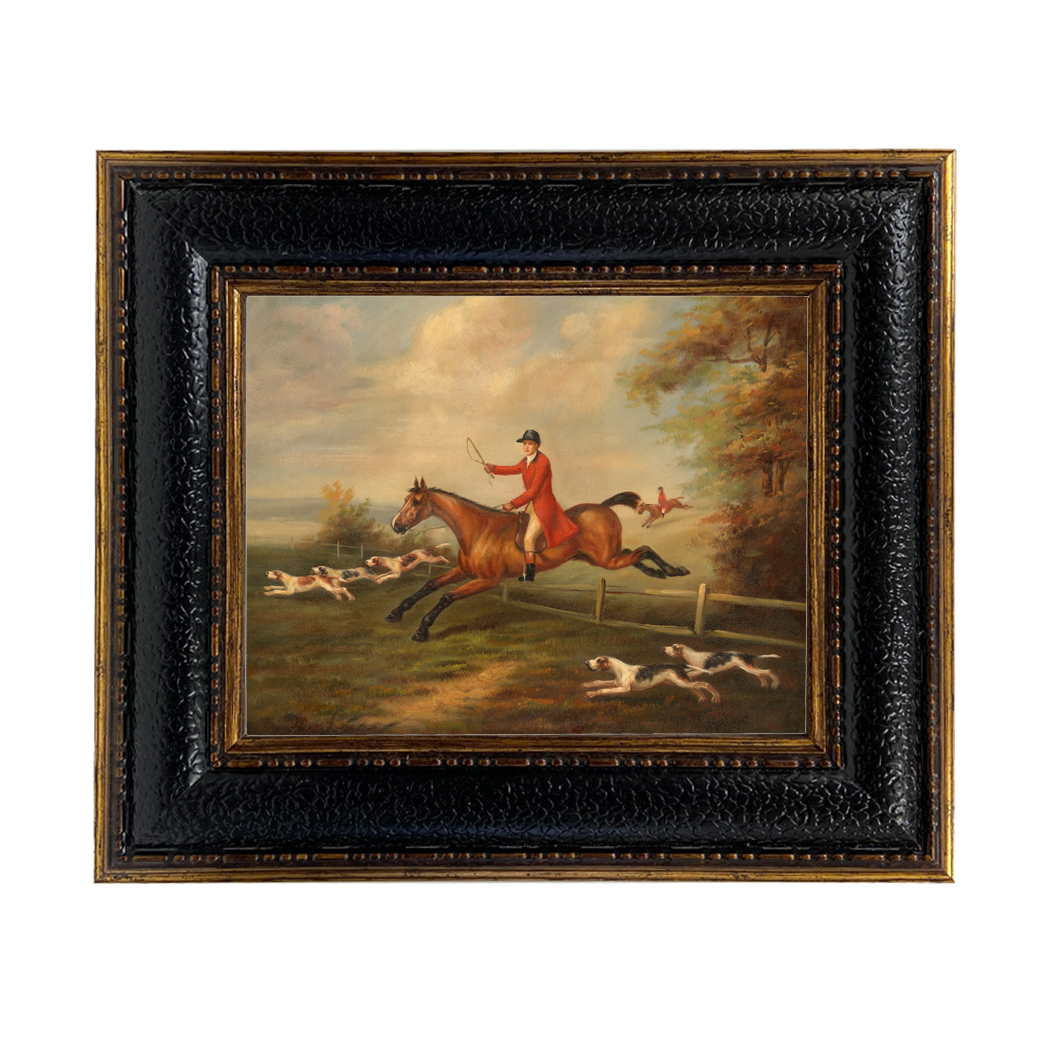This framed painting, encased in a thick, textured leather frame with gold trim, depicts an old-fashioned British hunting scene set in the countryside. At the center of the composition, a gentleman rider, clad in a long red riding coat, white trousers, and a black hunting cap, is captured in mid-jump as his brown horse with black hooves and tail clears a fence. The rider grips a riding crop in one hand and the horse's bridle in the other. Flanking the horse are five white hunting dogs with black spots, reminiscent of beagles, three on one side and two on the other. The background features a cloudy blue sky with scattered trees and a mix of grassy and bare dirt terrain. In the distance, another similarly dressed rider adds depth to the scene. The painting evokes a distinctly British, historical ambiance, thought to be from the 17th or 18th century.